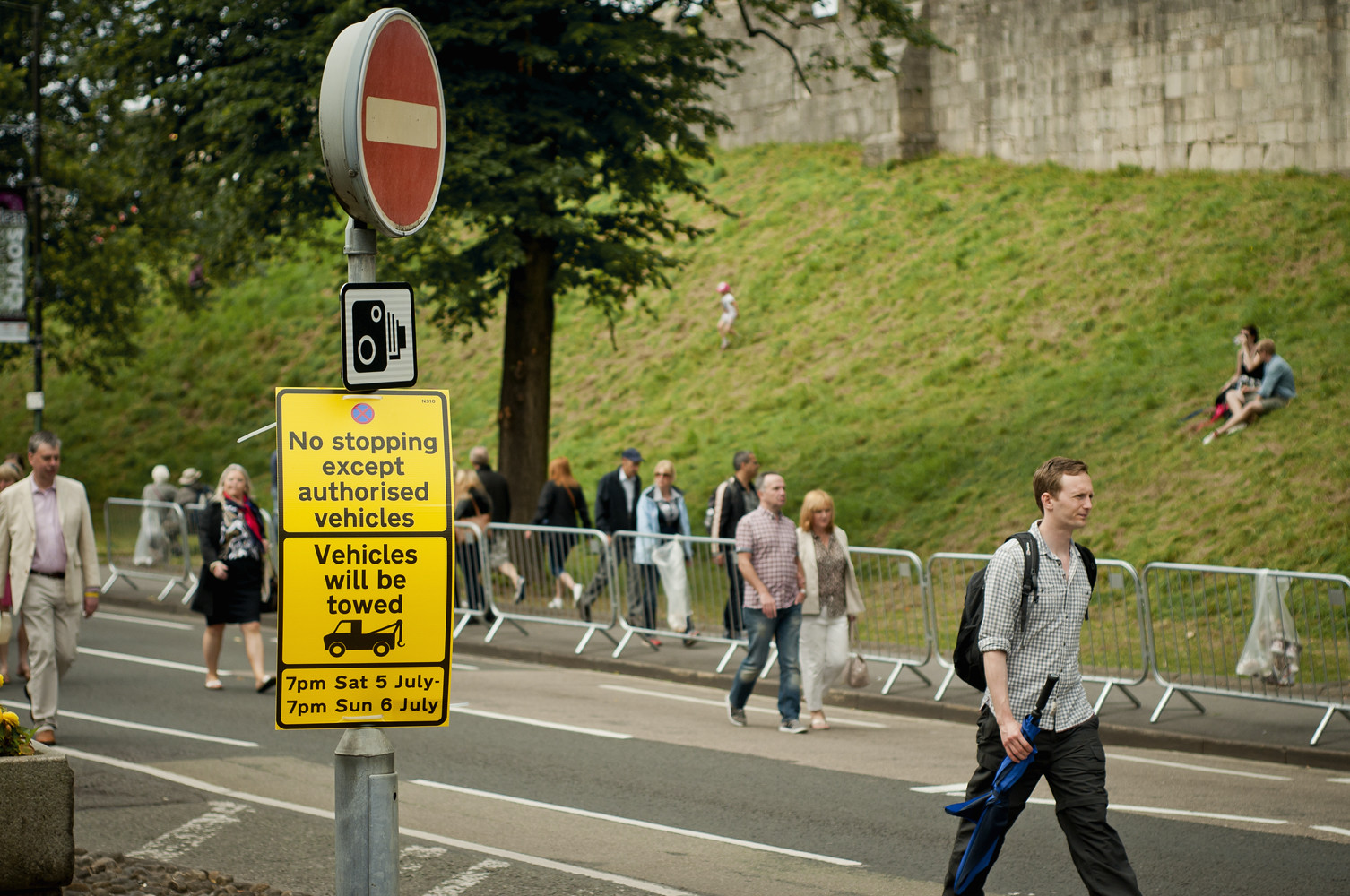In this color photograph, people are seen walking along an asphalt, two-lane road with white pavement lines, heading predominantly from the left side of the image to the right side. A man in the foreground, carrying an umbrella and wearing a backpack, is among the pedestrians. The road features a prominent yellow sign on a post to the left, reading "No stopping except authorized vehicles. Vehicles will be towed," along with the specific times and dates: 7 p.m. Saturday, 5th of July to 7 p.m. Sunday, 6th of July. Mounted above this is a red circular sign with a white bar through it, and a white sign with a black camera logo.

The street is lined with movable metal barricades on one side, beyond which lies a bustling sidewalk with numerous people walking in various directions. Adjacent to the sidewalk is a steep grassy slope, where several individuals are seated, and a child can be seen running down. The slope is bordered at the top by a gray concrete retaining wall and a green tree is visible to its side. Another tree stands on the left side of the image, adding to the greenery. The scene is vibrant and lively, capturing the collective movement and activity during the daytime.